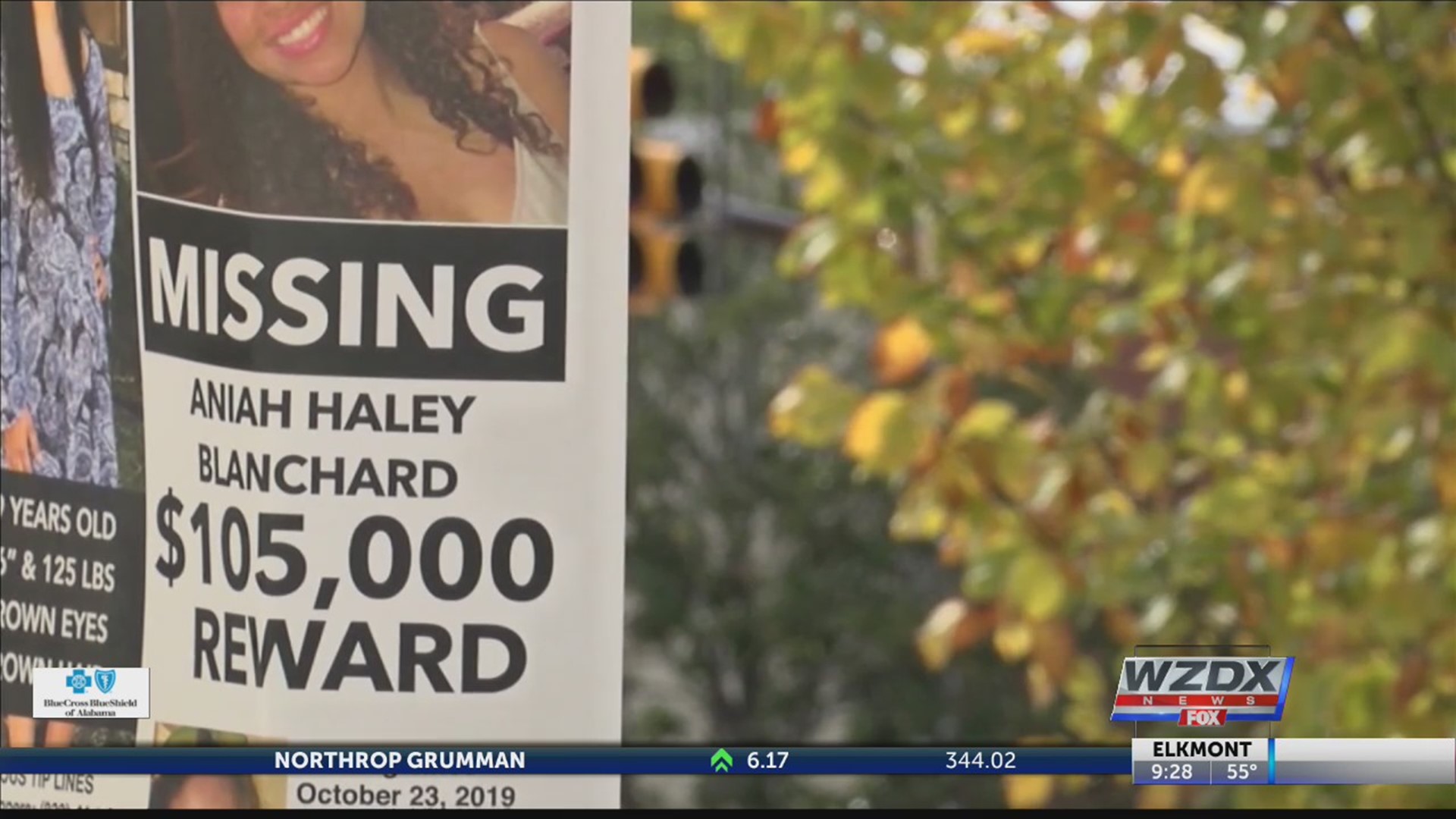This image is a detailed screenshot from a WZDX News segment on FOX News, dated October 23rd, 2019. The main focus is a missing person poster featuring Aniyah Haley Blanchard, with a reward amount of $105,000. The poster, showing a photo of the young woman and details such as age, weight, and eye color, appears attached to a wall or post. In the background, there is a blurred image of greenery and trees. Additional elements on the screen include stock market updates, specifically for Northrop Grumman, which is up by 6.17, totaling $344.02. The weather is also covered, with Elkmont displaying a current temperature of 55 degrees.